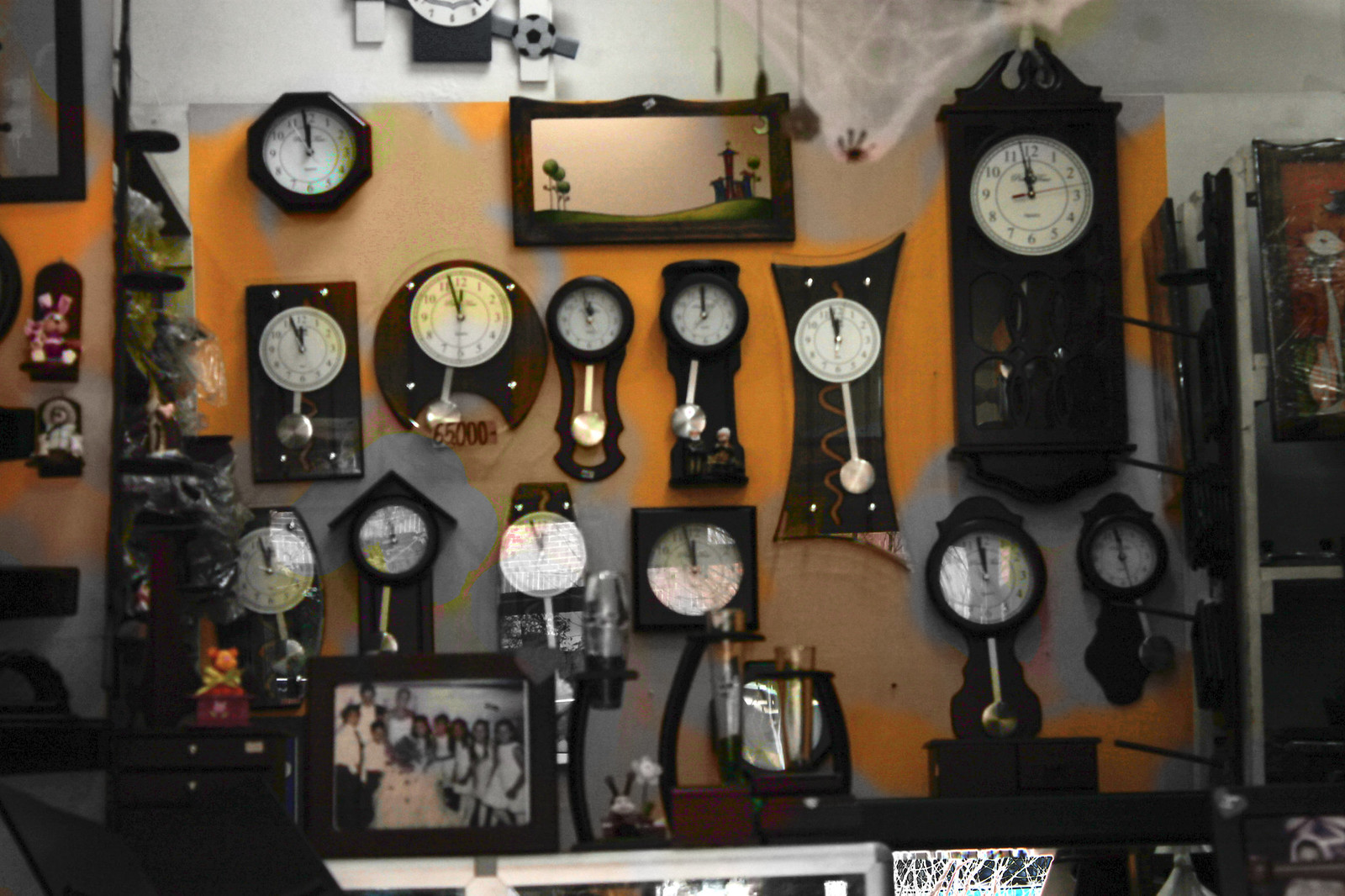In the color photograph, a gray and orange wall is adorned with a diverse collection of clocks, arranged neatly in rows. Most clocks feature white or off-white faces with black or dark brown outlines, and display either Roman numerals or regular numbers. The designs vary: some clocks are circular, others are square, and a few resemble small houses or ornate grandfather clocks with wooden cabinets and intricate details. Nearly all the clocks are set to around noon, though not perfectly synchronized, and many have silver pendulums hanging below their faces. Below this striking display, a table holds a framed photograph depicting a group portrait. In the picture, several girls, dressed in white dresses, are lined up alongside a couple of men in white shirts and dark ties. Additionally, a small Minnie Mouse figure is displayed on the wall, adding a whimsical touch to the scene.